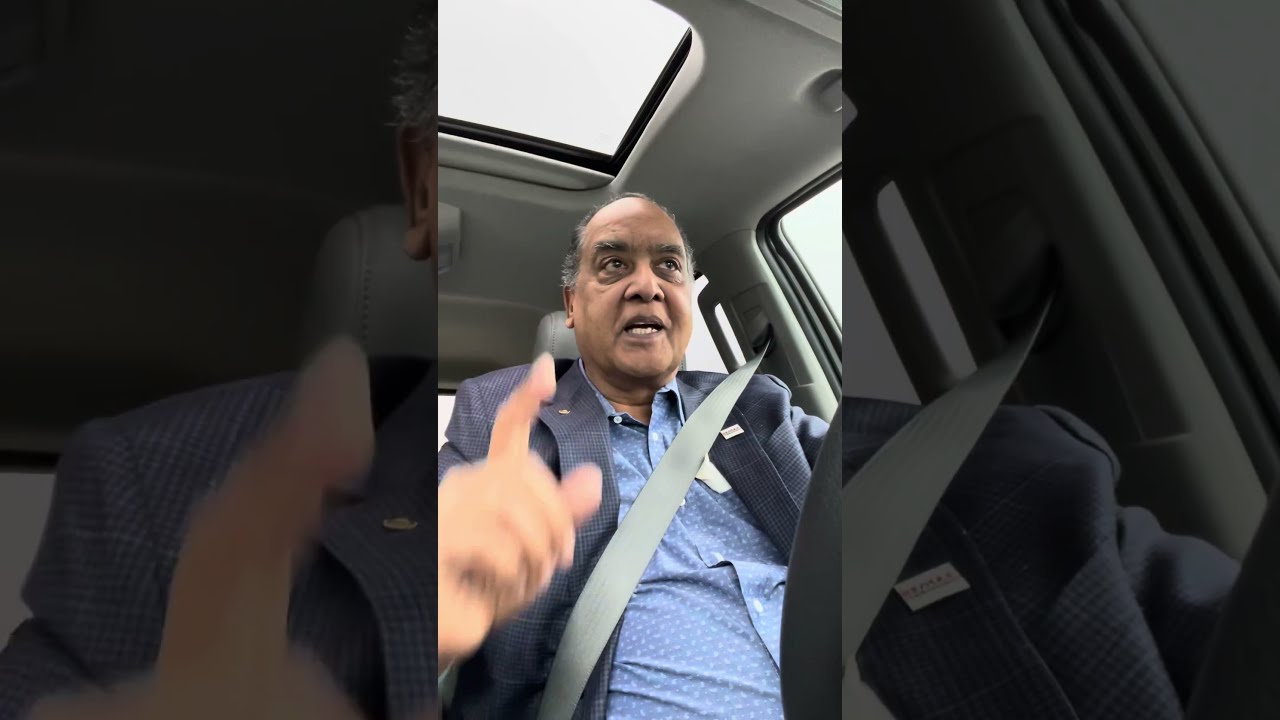This image captures an older gentleman, likely in his mid-50s, seated in the back of a car. The central figure, a man with brown skin and gray-black hair, is buckled in with a gray seatbelt. He is dressed in a stylish ensemble, featuring a gray, checkered patterned overcoat paired with a light blue, long-sleeve shirt adorned with white crosses. His mouth is slightly open as he gazes straight ahead. Above him, the car's visor is flipped up, and an open sunroof lets in light, revealing the roof's gray interior. The unique composition showcases this gentleman in the middle of the photo, flanked by two magnified and darkened sections of the image: an enlarged, up-close view of the side of his head to the left, and a darkened element of the car window's corner to the right. The visual focuses strongly on the centralized figure against the detailed backdrop of the car's interior.